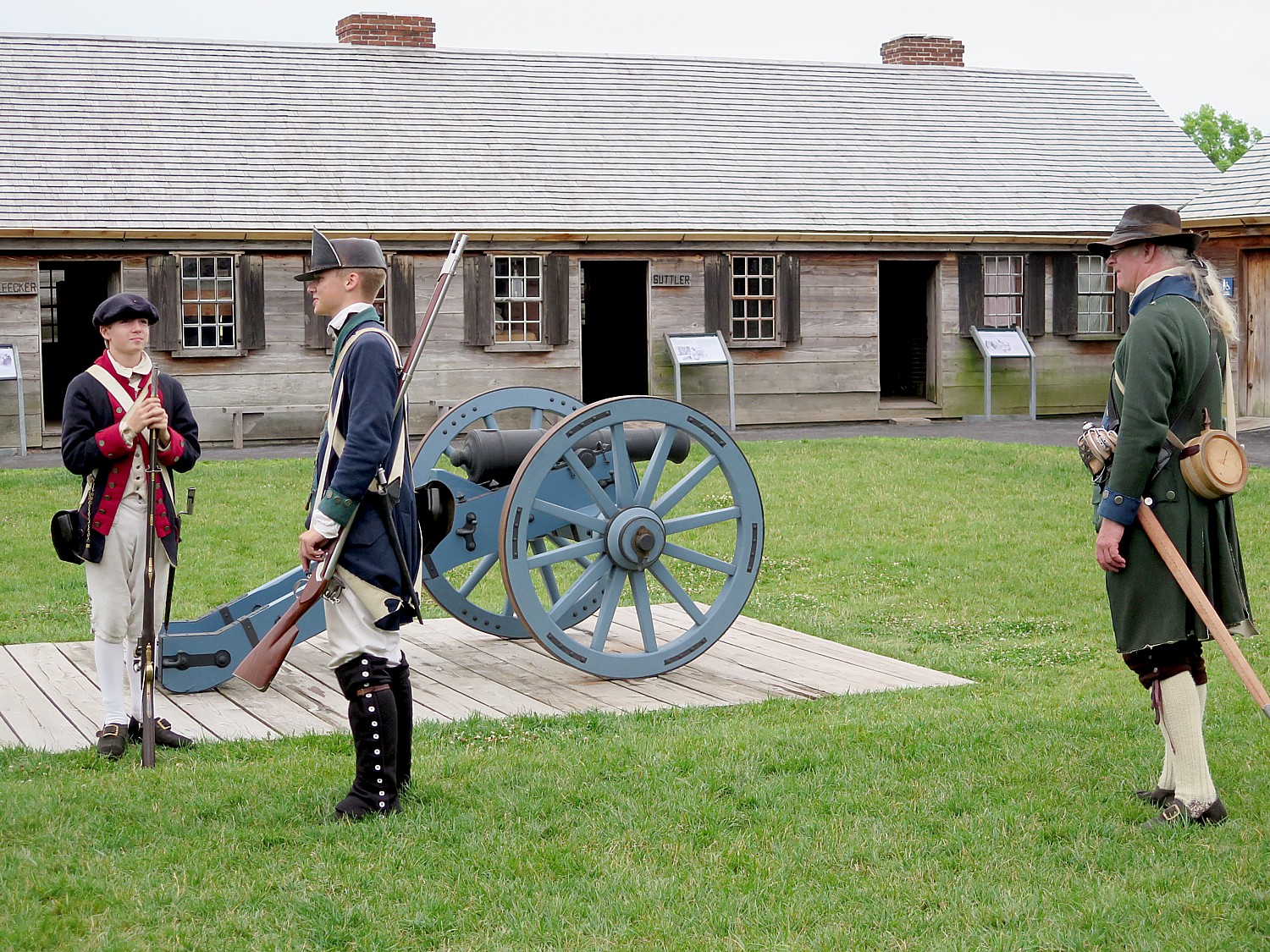This color photograph, taken outdoors, captures a scene steeped in history. Central to the image is a striking blue and black cannon set on a flat wooden plank platform, surrounded by lush green grass. The cannon, with its large blue wheels partially obscuring its barrel, is pointed to the right. Standing to the left in front of the cannon are three young men dressed as Revolutionary War reenactors. The soldier on the far left wears a blue jacket with red cuffs, light-colored pants, and a beret, carrying a musket. To his right is another soldier in a blue jacket with green trim, white pants, and black boots, also holding a musket. The third soldier, positioned further to the right, dons a green jacket with blue trim, a brown hat, and carries a sword, along with a canteen slung over his back.

In the background, an age-worn wooden building dominates the scene, its horizontal slats evoking a bygone era. The structure, marked with a plaque that reads "Suttler," features weathered wood, a pitched shingle roof, several chimneys, and at least three doors and four windows visible. Another similar building, possibly a bathroom, can be seen further to the right. Adding to the authenticity, signs on small stands are positioned beside the doors, underscoring the historic nature of the site.